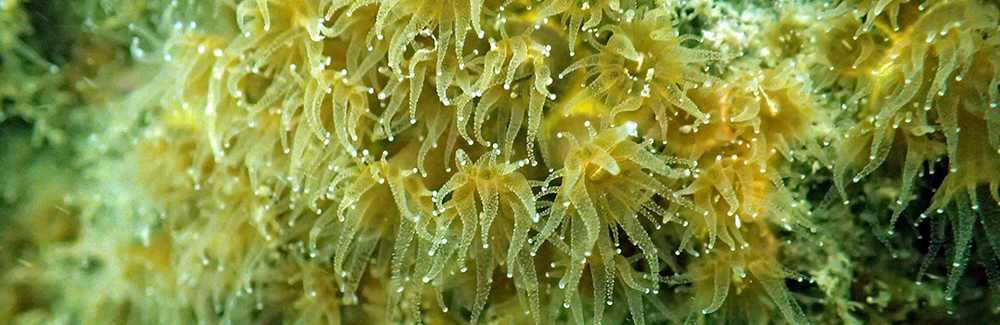This is a close-up image of a sea creature, most likely a sea anemone, characterized by its numerous tentacles. The dominant color in the image is a translucent yellow, which becomes clearer with a hint of green towards the tips of the tentacles. Each tentacle is capped with a small white sphere, and there are hundreds of these tentacles extending outward. The background is darker, suggesting the use of a flash in the photograph. The shape and arrangement of the tentacles create the impression of a singular organism, although the possibility of multiple creatures packed together cannot be ruled out. The image has a rectangular, horizontal layout and emphasizes the vivid, intricate details of the sea anemone’s tentacles against a blurred, darker background. The overall colors in the image range from yellowish-green to white, enhancing the appearance of an underwater sea creature.